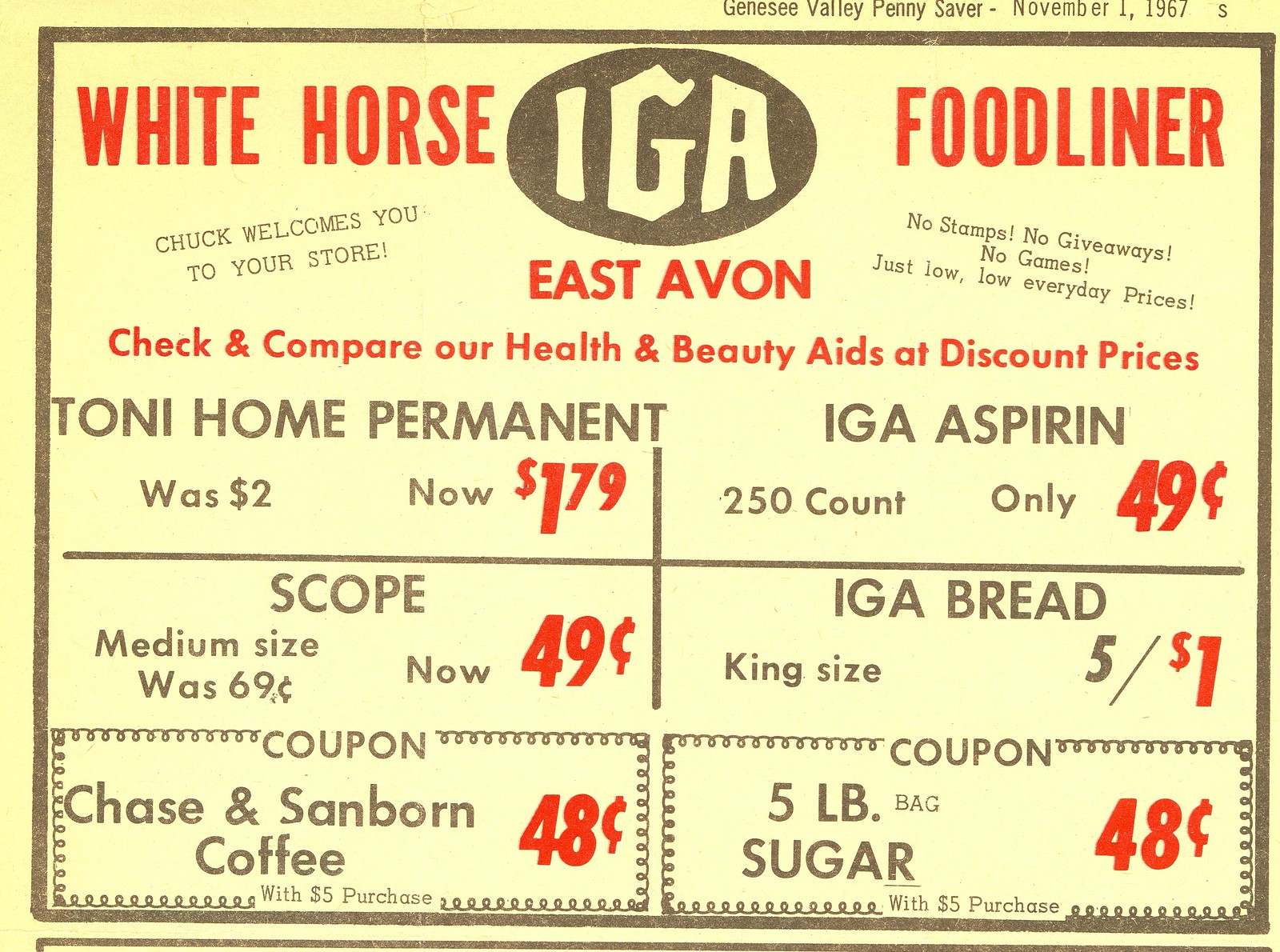This is a scanned image of a vintage store flyer dated November 1st, 1967, from the Genesee Valley Penny Saver. The flyer prominently features the 'White Horse' and 'IGA' logos, with 'Food Liner' in red font beside them. At the top right corner, 'Chuck welcomes you to the store' is written in small black font alongside the tagline, "No stamps, no giveaways, no games, just low, low everyday prices."

Centered on the flyer, in bold red uppercase letters, 'East Avon' is displayed. The flyer then encourages shoppers to "Check and compare our health and beauty aids at discount prices." Detailed below are several advertised deals: 
- Tony Home Permanent was $2, now $1.79
- IGA Aspirin, 250 count, only $0.49
- Scope, medium size was $0.69, now $0.49
- IGA Bread, king size, 5 for $1
- Chase and Sanborn Coffee, $0.48 with a $5 purchase
- Five Pound Bag of Sugar, $0.48 with a $5 purchase

The flyer features a mainly black, yellow, and red color scheme, with its content well-spaced across the entire page for clear visibility of the promotions and logos.